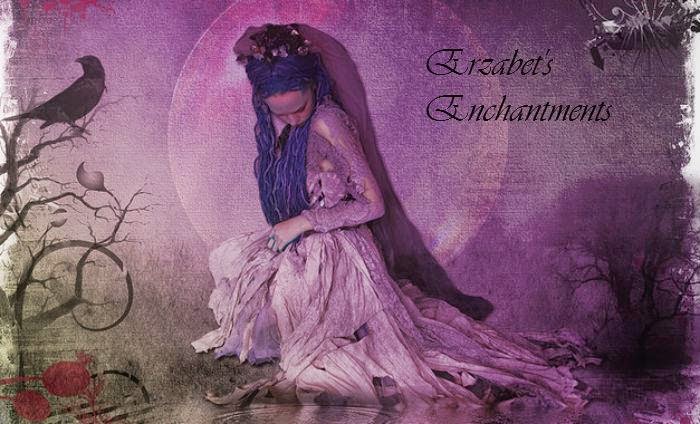The image appears to be a detailed, digitally created or painted scene, possibly resembling an advertisement or the cover of a postcard. Central to the composition is a woman with long, dark purple hair sitting down, dressed in a purple gown with white tones. She is gazing downward, focused on her dress. Her facial features are partly obscured except for her forehead and nose. 

In the background, there's a large, pinkish-purple moon that adds a mystical ambiance to the setting. To the left of the woman, a dried-out tree with a single bird, likely a crow, is depicted, bringing an element of nature into the scene. The predominant color scheme includes various shades of purple, pink, gray, red, and black, contributing to a dreamlike, enchanting atmosphere.

In the upper right corner of the image, the text "Elizabeth's Enchantments" is prominently displayed in black letters, suggesting a magical or fantasy theme for the piece. The overall style is artistic and visually captivating, suitable for an advertisement or a whimsical postcard.